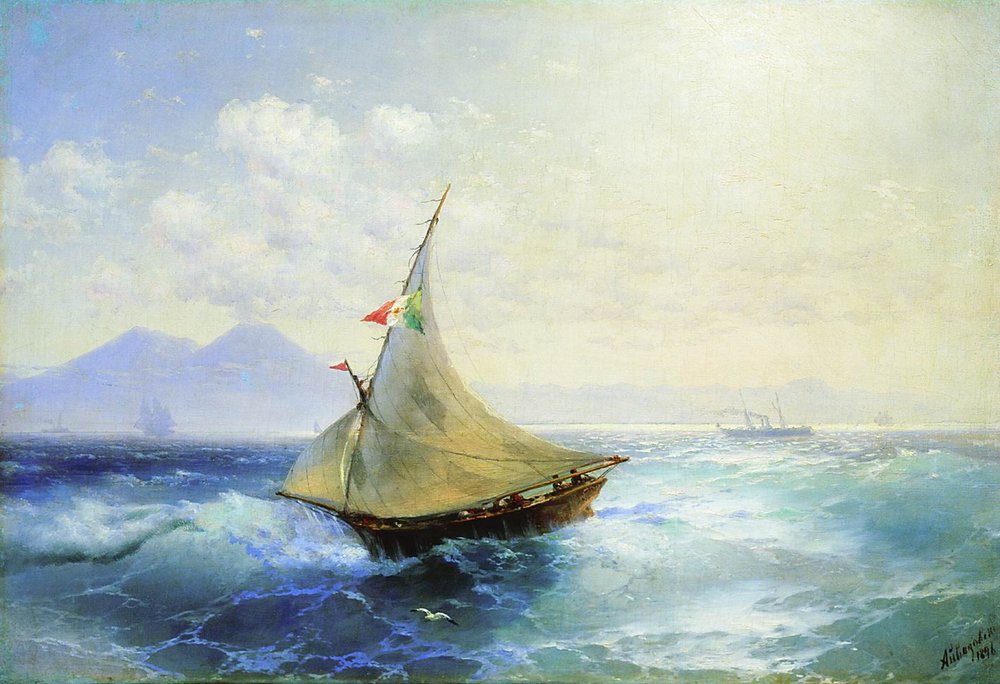The painting depicts a sailboat navigating a choppy ocean, where waves vary from dark blue on the left to light blue on the right, topped with white foam. The sailboat, crafted from wood brown, stands prominently in the center foreground. Its triangular white sails are currently unfolded, displaying a red, white, and green flag, indicative of the Mexican flag, hanging from the mast. Human figures are visible on the boat, adding life to the scene. Beyond this primary vessel, several gray ships are faintly visible, their details obscured by distance. The horizon features jagged, bare mountains, one of which is actively spewing white smoke from its peak. The sky above transitions from a clear light blue at the top to a paler, almost white shade as it approaches the horizon. Scattered fluffy white clouds hover mid-sky. The vivid scenery captures a snapshot of nautical life against a dramatic and serene backdrop.